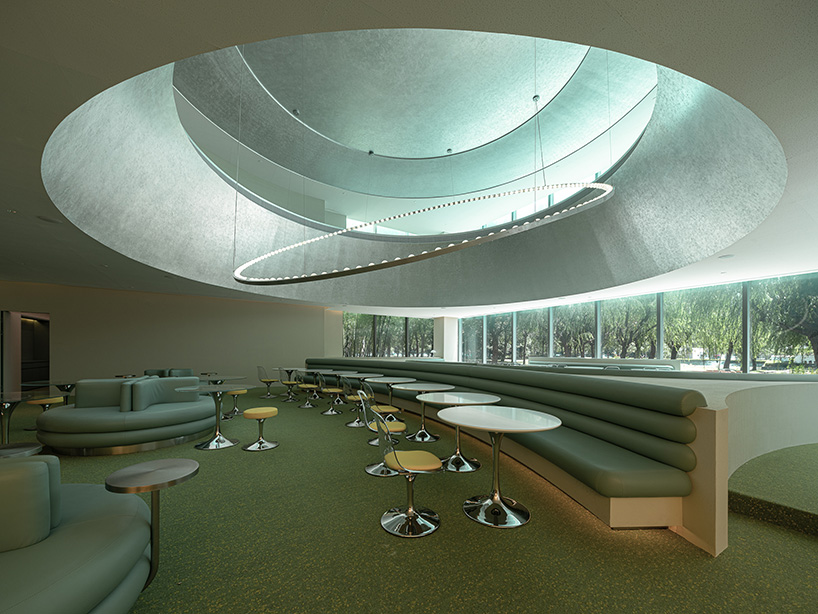The image depicts a modern open-space lounge area with a notable architectural feature—a large circular skylight in the ceiling that juts upward, creating an effect of higher ceilings. Hanging from this skylight is a tilted circular light fixture adorned with numerous lights, suspended by wires. The floor is carpeted in a dark green hue.

Within the room, various seating arrangements are visible. On one side, there's a long bench with white cocktail tables positioned in front of it, each accompanied by a single metallic chair with orange (or possibly dark yellow) cushions. Toward the center, circular sofas are arranged with tables placed in every indentation, each table partnered with a cushioned metal chair. 

A wall at the back of the room is lined with a continuous row of windows that allow natural light to permeate the space, offering a view of the trees outside. Additionally, scattered throughout the room are more metallic chairs with dark yellow cushions. Near the left side of the room, a door is visible. This meticulous setup, featuring a combination of circular sofas, long benches, and metallic chairs, underscores the room's modern and sophisticated ambiance.